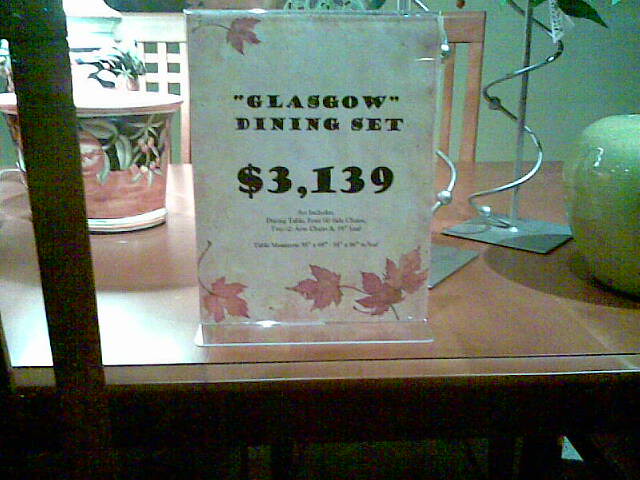The image shows a Glass Glow Dining Set priced at $3,139, prominently displayed on a light wood dining table. The table is adorned with decorative fall-themed maple leaves and assorted objects, including a green glass apple-shaped ornament on the right, a potted plant with green and red leaves, and a spiraling metal decoration. The dining table is part of a set that also includes wooden chairs, one of which is partially visible in the background. The image itself appears grainy and is seen through a clear plexiglass barrier that frames the scene, giving it an almost resale feel despite the elegant setup. The table's surface holds a mix of decor that hints at both new and possibly gently used items.